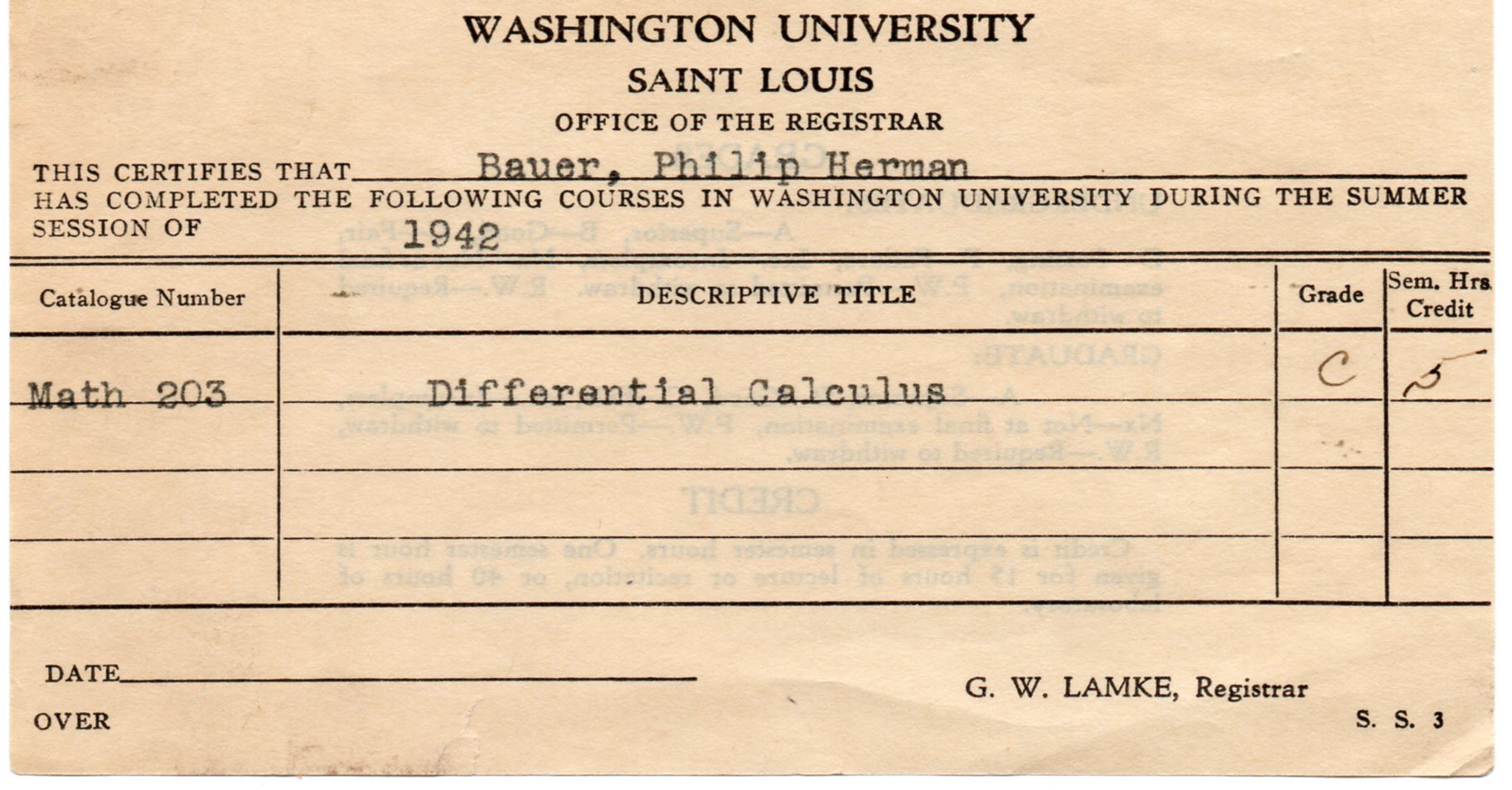The image showcases a vintage, cream-colored document from Washington University in St. Louis, specifically from the Office of the Registrar. The black text at the top is centered, reading "Washington University," with "St. Louis" below it, followed by "Office of the Registrar." The document certifies that "Bauer, Philip Herman" has completed coursework during the summer session of 1942. It lists the course "Math 203 - Differential Calculus," for which a grade of "C" was earned with 0.5 semester hours of credit. Positioned in a columnar table, the headings include "Catalog Number," "Descriptive Title," "Grade," and "Semester Hours Credit." The form includes a line for the date, which remains blank, and at the bottom right, the typed name "G.W. Lemke, Registrar." The document has aged, giving the paper a tannish, cream tone with black text. The layout is landscape orientation, and it appears to be a photograph of a certificate proving completion of a differential calculus course.